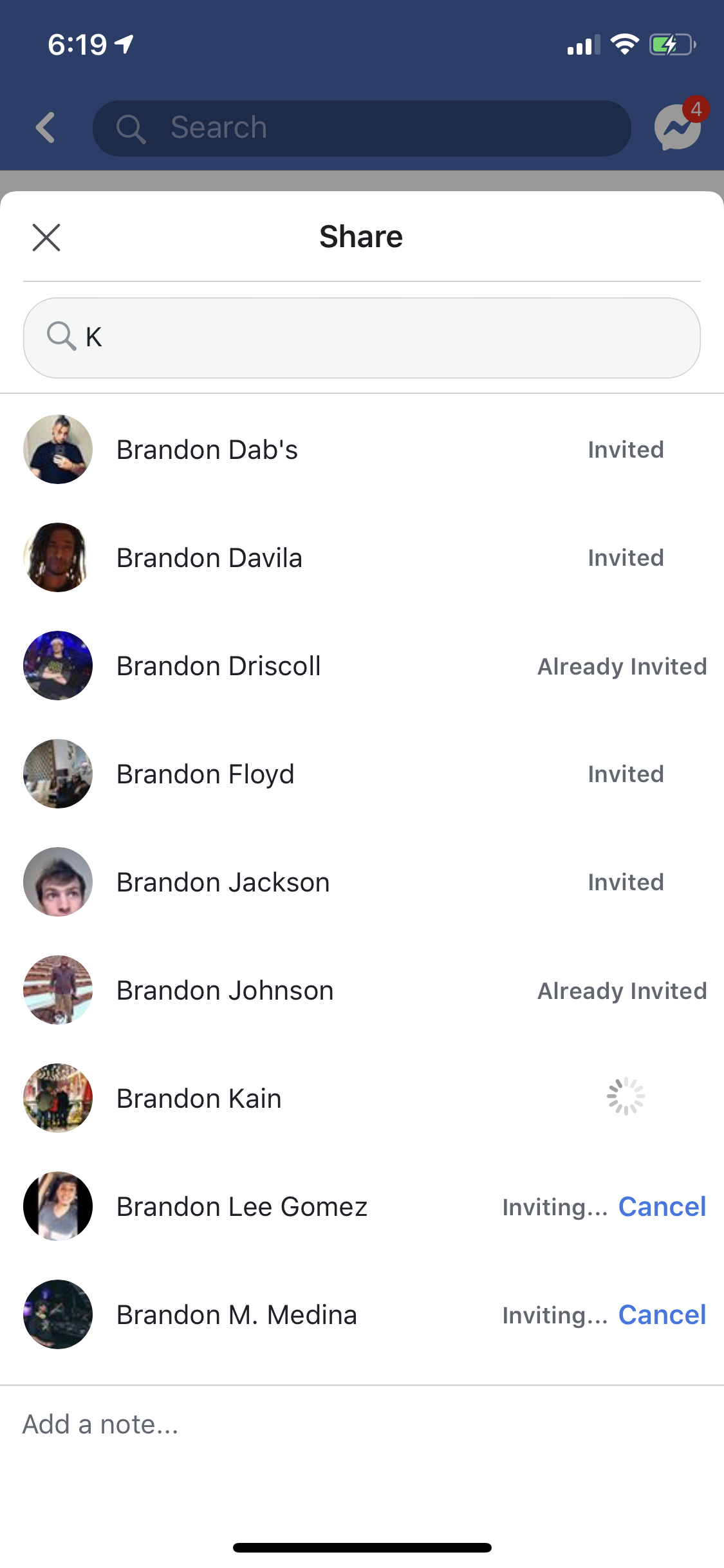This is a detailed screenshot of a phone's screen with a dark blue or black border at the top displaying the time as 6:19. The status bar shows a green battery icon indicating the phone is halfway charged, and the Wi-Fi signal has three bars with four messages waiting to be read. Below this, the word "share" is clearly visible, followed by a search bar containing the letter "K" with a magnifying glass icon to its left. Underneath, a list of nine names with corresponding profile pictures is displayed vertically. Each person is named Brandon with different last names, including Brandon Dabbs, Brandon Davila, Brandon Driscoll, Brandon Floyd, Brandon Jackson, Brandon Johnson, Brandon Kane, Brandon Lee Gomez, and Brandon M. Medina. To the right of each name, it indicates their invitation status: "invited," "already invited," "inviting," with Brandon Kane showing a loading circle, and Brandon Lee Gomez and Brandon M. Medina showing "inviting" alongside three dots and the option to "cancel" in blue text. The bottom of the screen features a dark blue or black line, with the option to "add a note" just above it.